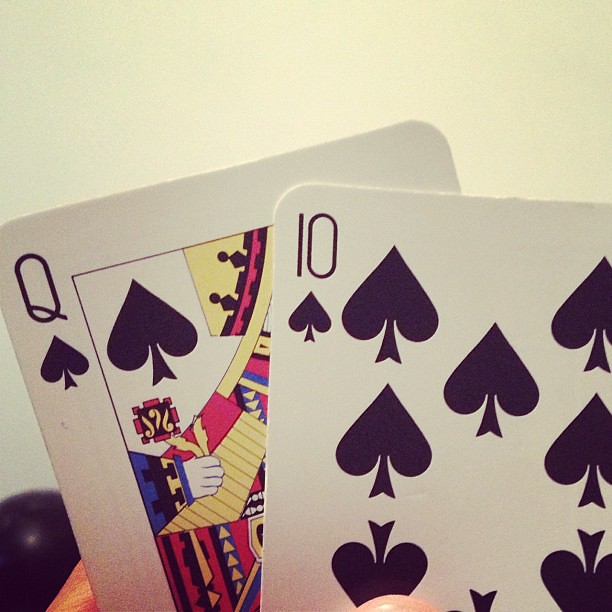In the foreground, dominating approximately 75% of the image, two playing cards—a Queen of Spades partially covered by a 10 of Spades—are held in what appears to be a pair of hands. The scene is set against a white wall and, further back, a possibly black exercise ball. The cards belong to a standard deck, showing signs of use, evidenced by a slight smudge near the top left corner of the Queen of Spades, just below the "Q" and spade icon. The owner's thumb and the backs of their hands are visible, hinting at a possible card game, though the exact game and player's intentions remain unclear.